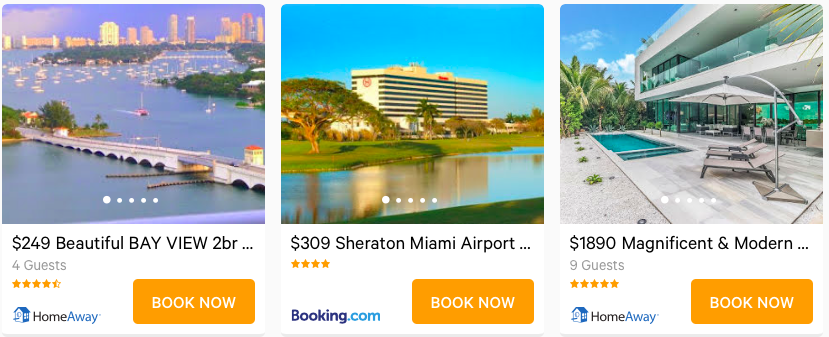This screen capture from a vacation rental website showcases various properties available for booking. On the left, there's an image depicting a serene bay surrounded by numerous buildings, likely located in Florida. Below this image, the listing shows a price of $249 per night for a "Beautiful Bay View" condominium, which includes two bedrooms and accommodates up to four guests. The property boasts a rating of four and a half stars and is listed under "HomeAway," accompanied by a home icon and a "Book Now" button.

Adjacent to this, there is a listing for the Sheraton Miami Airport Hotel priced at $309 per night. The hotel's image is displayed above its listing, which features a four-star rating and a "booking.com" label next to an orange "Book Now" button.

On the right side, the capture features a listing for a "Magnificent and Modern View" property, priced at $1,890 per night. This luxurious option can host up to nine guests and has earned a five-star rating. It is also listed under "HomeAway," with an accompanying home icon and an orange "Book Now" button. The image for this listing shows a beautifully maintained condo or house with a scenic backyard.